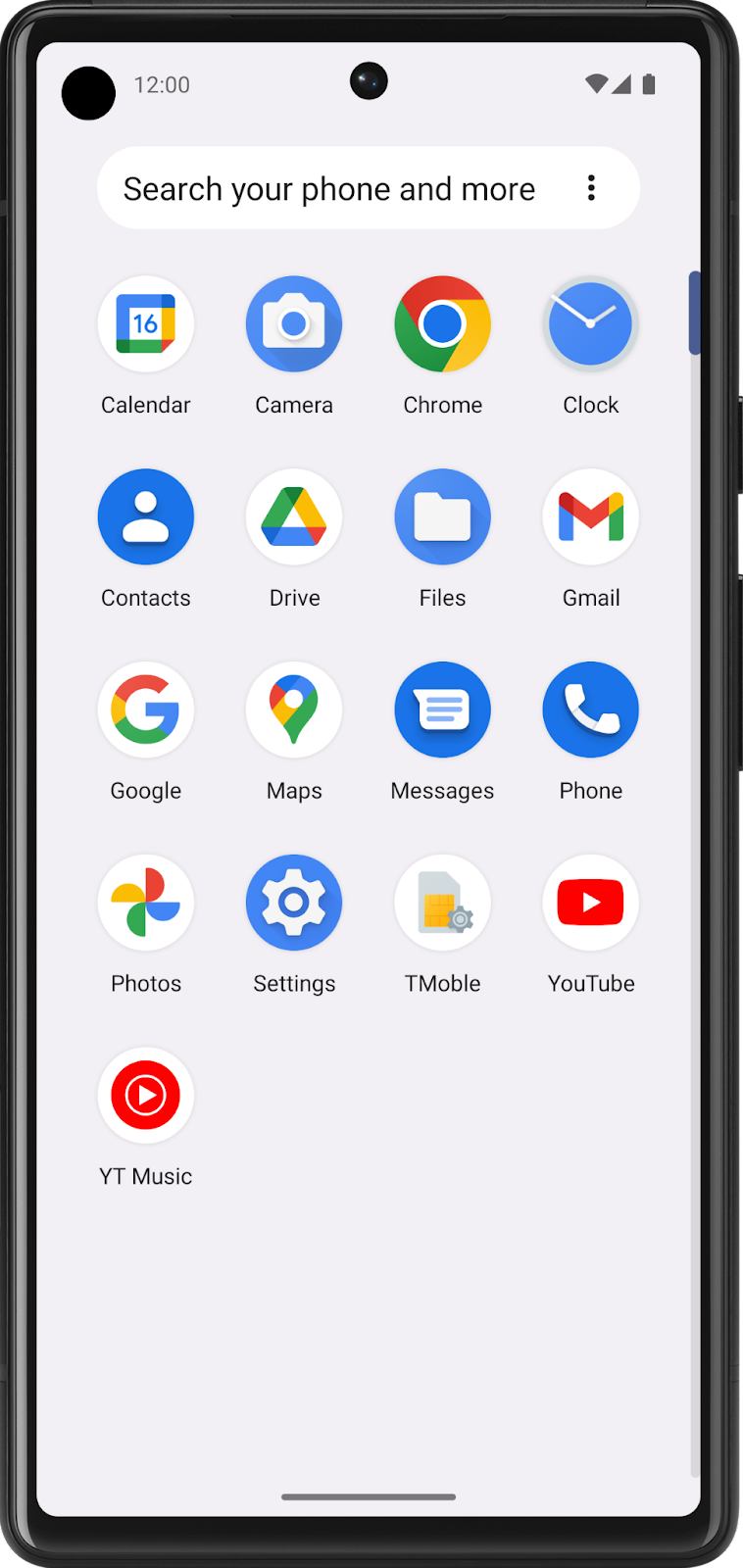A close-up image depicts a smartphone screen displaying a variety of app icons with their corresponding labels. At the top of the screen, the time is clearly shown as 12:00. Just below the time, there is a search bar with the placeholder text "Search your phone and more."

The screen is populated with numerous app icons, each with a distinct design and label:
1. **Calendar** - An icon depicting a calendar.
2. **Camera** - An image of a camera.
3. **Chrome** - The Google Chrome logo with "Chrome" written underneath.
4. **Clock** - An icon of an analog clock.
5. **Contacts** - A blue circle featuring a basic person outline.
6. **Drive** - A rainbow-colored triangle representing Google Drive.
7. **Files** - An icon of a folder.
8. **Gmail** - A colorful 'M' symbolizing Gmail.
9. **Google** - A colorful 'G' for the Google app.
10. **Maps** - A pin drop icon in Google’s signature colors for Google Maps.
11. **Messages** - An icon resembling a piece of paper with lines.
12. **Phone** - A classic telephone icon.
13. **Photos** - A pinwheel icon representing Google Photos.
14. **Settings** - An icon of a gear.
15. **T-Mobile** - An unrecognized symbol associated with T-Mobile.
16. **YouTube** - A red play button symbol for YouTube.
17. **YouTube Music** - A circular red play button for YouTube Music.

This image offers a detailed view of various app icons on a smartphone screen, providing quick access to essential functions and services.